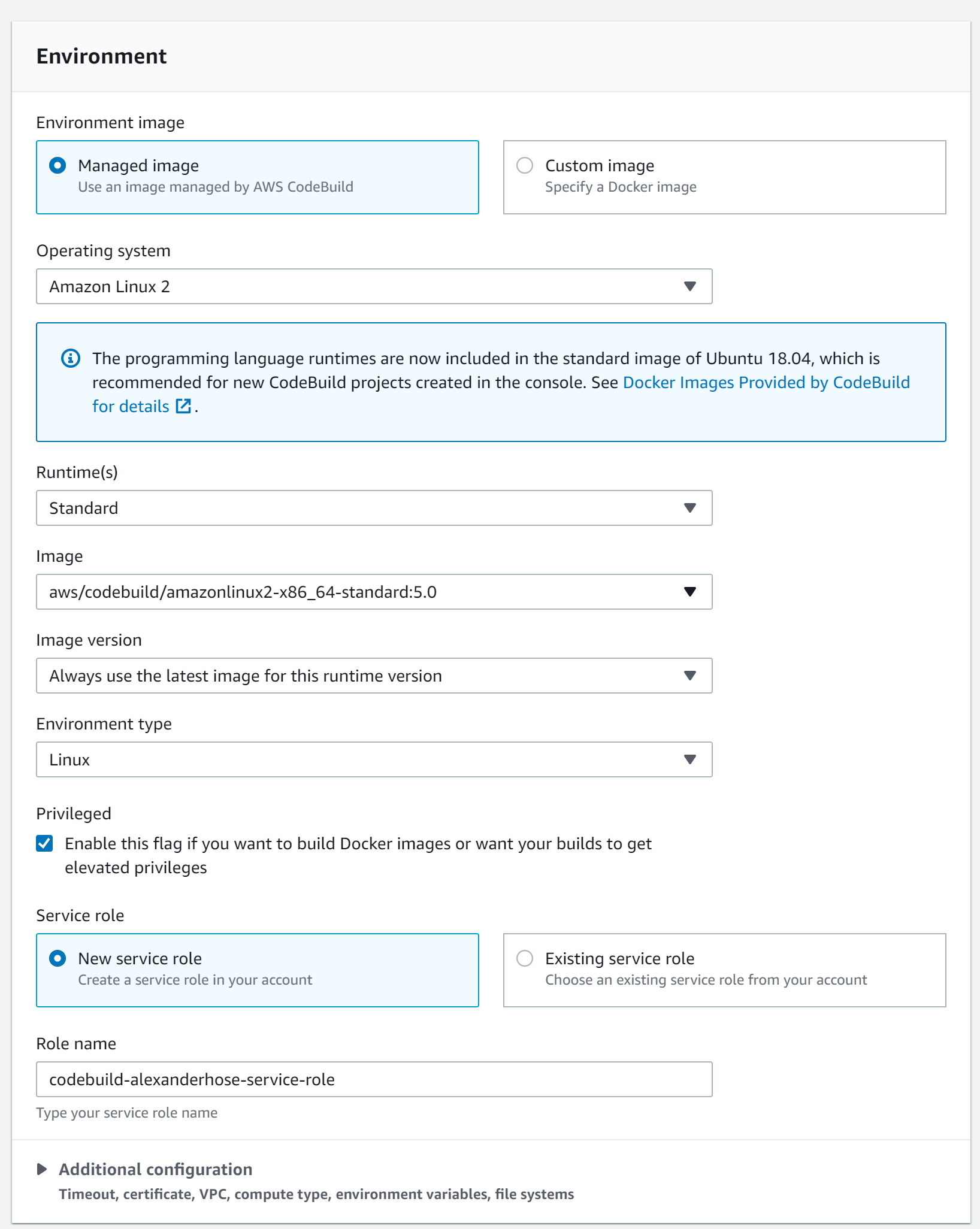**Caption:**

This image captures a detailed screenshot from a website interface designed for configuring an environment setup, presumably related to AWS CodeBuild. The screenshot features a medium to light gray border surrounding the entire layout.

At the top of the interface, there is a prominent dark black text banner labeled "Environment," with the word "Environment" in capitalized letters.

Below this, the main section of the page features a white background with the heading "Environment Image." Included within this section is a blue-bordered rectangular box with a blue background. Inside this rectangle, there is a dark blue circular button labeled "Managed Image," which indicates an option to use an image managed by AWS CodeBuild. 

Additionally, there is an alternative radio button option labeled "Custom Image," allowing users to specify a Docker image; however, this option is not selected and is depicted as a white-centered circle.

Further down, the "Operating System" section is shown with "Amazon Linux 2" as the selected option, accompanied by a drop-down menu for other potential choices. 

A blue informational banner follows, containing a message regarding programming language runtimes. The banner informs users that these runtimes are included in the standard image of "Ubuntu 18.04," recommended for new CodeBuild projects created in the console. It also prompts users to see Docker images provided by CodeBuild for detailed information.

Subsequently, the "Run times" section is presented with a drop-down menu set to "Standard." This is followed by the "Image" section with its respective drop-down menu, indicating the image version setting to "Always use the latest images for this run time version."

The "Environment Type" section shows "Linux" with another drop-down menu to possibly select other types. The "Privileged" option is checked, emphasizing that enabling this flag allows the building of Docker images or grants elevated privileges for the builds.

Lastly, the "Service Roles" section provides options for "New Service Role" or "Existing Service Role," with "New Service Role" currently chosen. The screenshot includes fields for "Role Name" and "Additional Configuration," hinting at advanced settings for further customization.